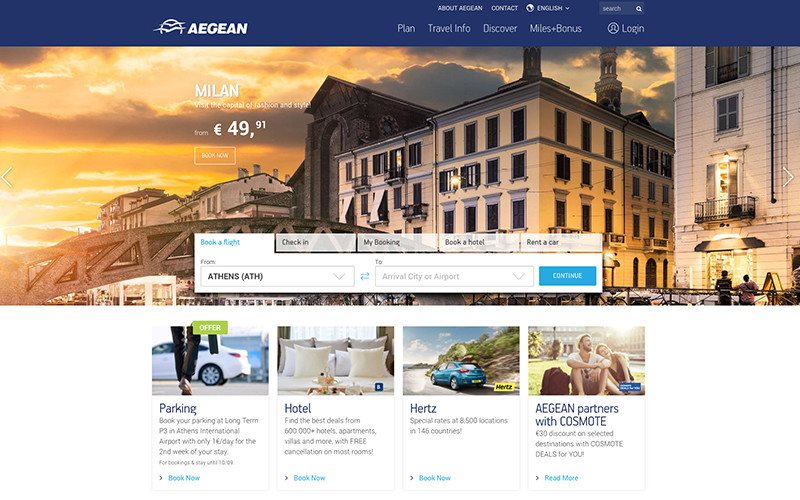Screenshot of the Aegean Airlines Travel Website

The screenshot captures the Aegean Airlines travel website's desktop interface. At the top of the page, a dark navy blue bar features the distinctive white Aegean logo. Adjacent to the logo, a series of five light gray navigation menus are displayed: "Plan," "Travel Info," "Discover," "Miles+Bonus," and "Login." Above these menus is a minimalistic gray strip containing links for "About Aegean," "Contact," a language dropdown menu, and a small search box.

Dominating the main section of the webpage is a vibrant image, likely of Milan, showcasing a picturesque view of homes and businesses, each rising three to four stories high, with a bridge seamlessly connecting parts of the city. The background hints at an enchanting sunset scattered with clouds, creating a serene and inviting atmosphere.

Centered on this image is a prominent rectangular module designed for booking flights. It begins with a highlighted "Book a Flight" prompt in blue letters and provides fields starting with "From Athens (ATH)" followed by an input for the "Arrival City or Airport." A striking blue "Continue" button awaits user interaction. Below this booking module are unselected tabs for "Check-in," "My Booking," "Book a Hotel," and "Rent a Car."

Beneath the main image, the webpage shifts to a clean white background presenting four categorized sections side by side: "Parking," "Hotel," "Hertz," and "Aegean Partners with Cosmo." Each category features a small, representative image above it. The "Parking" category displays an icon of a person walking towards a car. Next, "Hotel" includes an icon of a bed adorned with pillows. The "Hertz" section showcases a blue car facing away from the viewer. Lastly, "Aegean Partners with Cosmo" highlights a heartwarming image of a man and woman sitting in a park, with the woman resting her head on the man's shoulder.

This comprehensive layout provides users with an intuitive navigation experience and all necessary tools to explore and book their travel seamlessly.